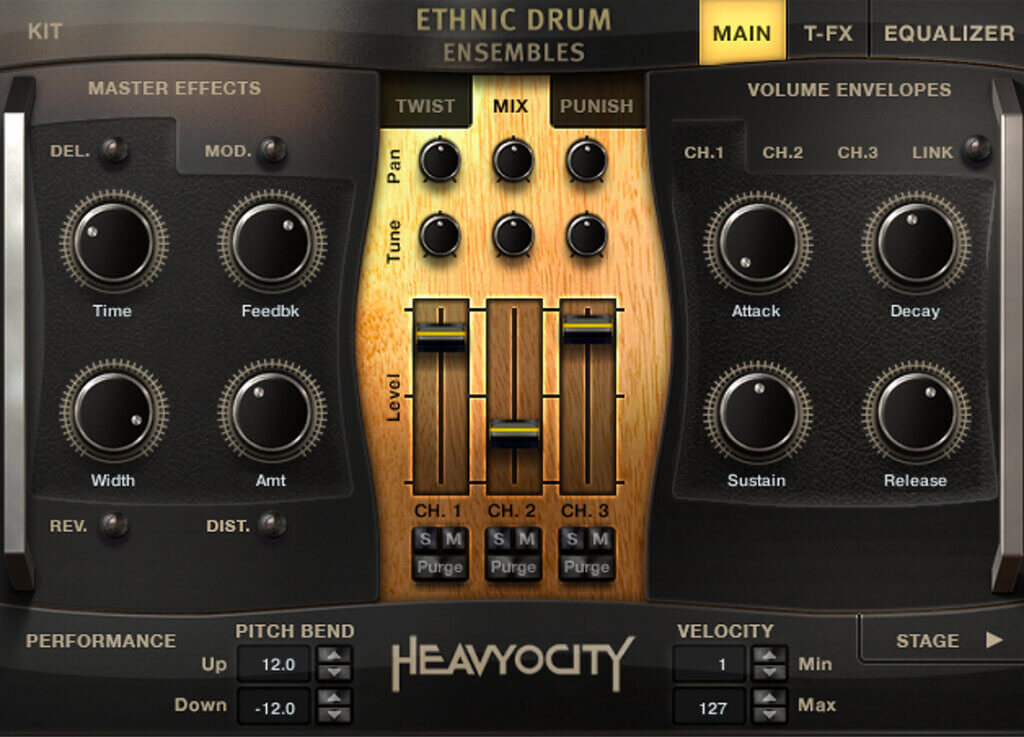This image depicts a digital interface for an audio equalizer, specifically designed to replicate the control panel of an ethnic drum ensemble, and appears to be a virtual drum machine app for a computer. At the top of the interface is the title "Ethnic Drum Ensembles" in brown text, with a smaller label, "Equalizer," in the upper right corner. To its immediate left is a lit-up "Main" button. 

The equalizer section is divided into two groups of four black rotary knobs. The left-hand group controls Time, Feedback, Width, and Amount, while the right-hand group handles Attack, Decay, Sustain, and Release. In the middle, there are additional control elements, including three vertical sliders that likely adjust various levels.

Additionally, the panel includes sections for Master Effects, Delay, Modulation, Reverb, Distortion, Twist, Mix, and a "Punish" function, indicating a comprehensive set of tools for audio manipulation. This app appears to visually mimic real-world audio equipment, down to the intricate details and varied control options. Notably, the product is labeled as being made by Heavyocity.